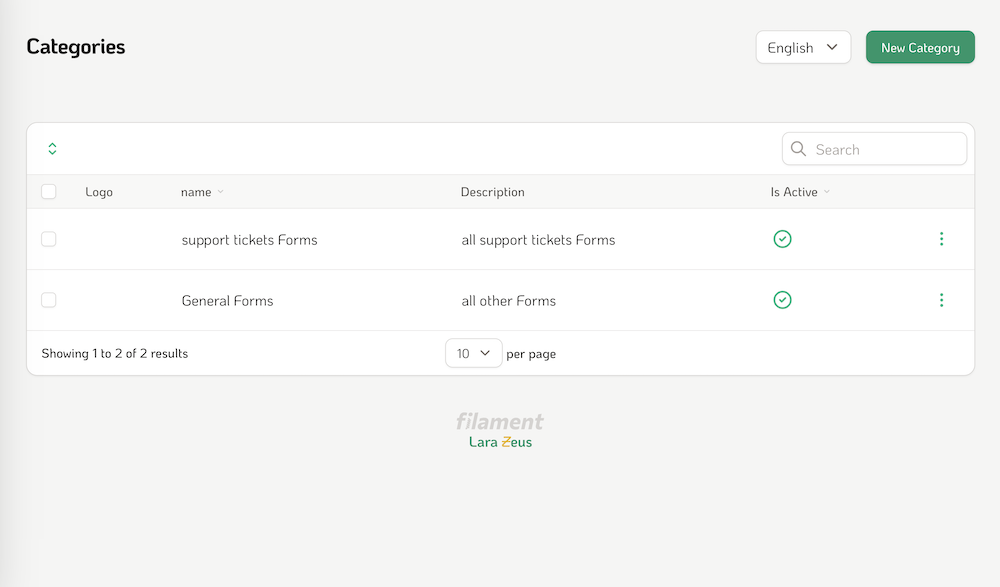The interface depicted in the image features a grey background with black text. In the upper left corner, there is a label that says "Categories." Positioned more towards the right, there's a drop-down box displaying the text "English" in white on a black background. Adjacent to this, a green button labeled "New Category" in white text is prominently placed.

Below this header section, the main content area consists of a white box with alternating white and grey lines, although only the first line is grey. On the upper left of this box, there are grey up and down arrows for sorting options. To the right, a white search box is situated. Along the grey line in this main content area, there's a white square on the left. Next to it, bold black text reads "Logo," "Name," "Description," and "Active."

The section beneath this describes two rows of entries. The first row includes: "Support Tickets Forms" and "Support All Tickets Forms" in white text. To the right of these labels, a green circle with a white checkmark, and three grey dots signifying additional options, are present. The second row mirrors this structure with the label "General Forms" and "All Other Forms," also accompanied by a green checkmark and three grey dots.

At the bottom left of these entries, black text states “Showing 1 of 2 results.” To the right of this, a drop-down menu offering the number "10" next to "Per Page" is present.

The footer of the interface has "Filament" written in grey, followed by "Laura Zeus" in black, except for a distinctive yellow "Z" with a European-style line through it.